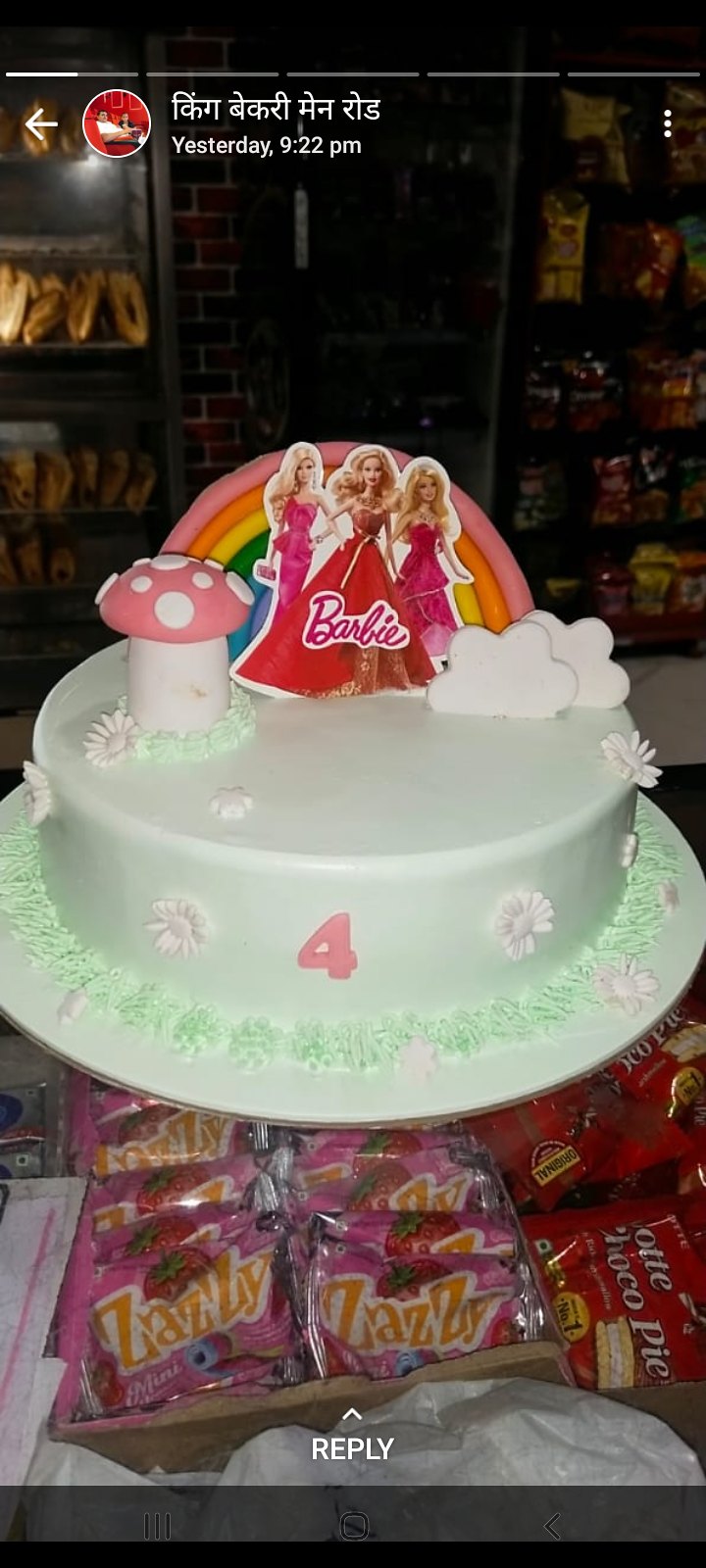The image is a screenshot of a phone display, capturing a photograph posted on social media at 9:22 PM, indicated by text in what appears to be an Indian script. The focal point is a birthday cake. The cake, adorned in smooth lime green fondant, features a prominent pink number 4 on the front, likely celebrating a fourth birthday. Detailed decorations include green frosting piped around its base, mimicking grass, and a distinct white-stemmed mushroom with a red cap and white dots on top. A central cutout of three Barbie dolls with the word "Barbie" amidst clouds and a rainbow is placed atop the cake. Surrounding the cake are various snacks, including "Choco Pie" and "Zazzy" candy, suggesting a festive setting. At the bottom of the screenshot, the word "Reply" is visible, emphasizing the social media interface.